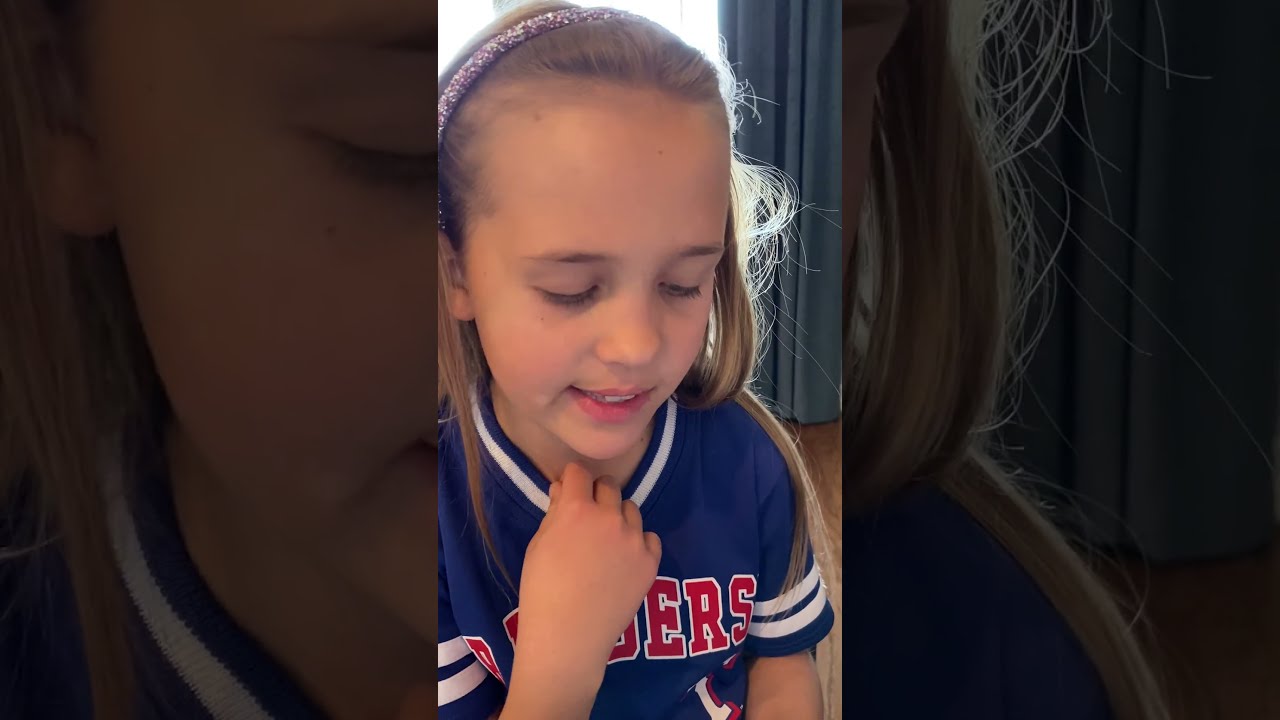The image is a horizontally rectangular three-paneled composition showcasing a repeated photograph of a young girl in a room. Each end panel displays a darkened close-up of the central image. In the central panel, the girl, who appears to be around seven or eight years old, has dirty blonde hair that extends past her shoulders and wears a sparkling hairband with purplish and whitish hues to keep her hair back. She is dressed in a blue sports jersey with white stripes on the sleeves and a white collar, detailed with red letters outlined in white, partially reading "ERS" as her hand covers the beginning letters. The girl is looking down, slightly smiling, and appears to be speaking, with one hand holding the neck of her shirt. The background reveals a wooden, brown floor and blue or steely gray curtains.